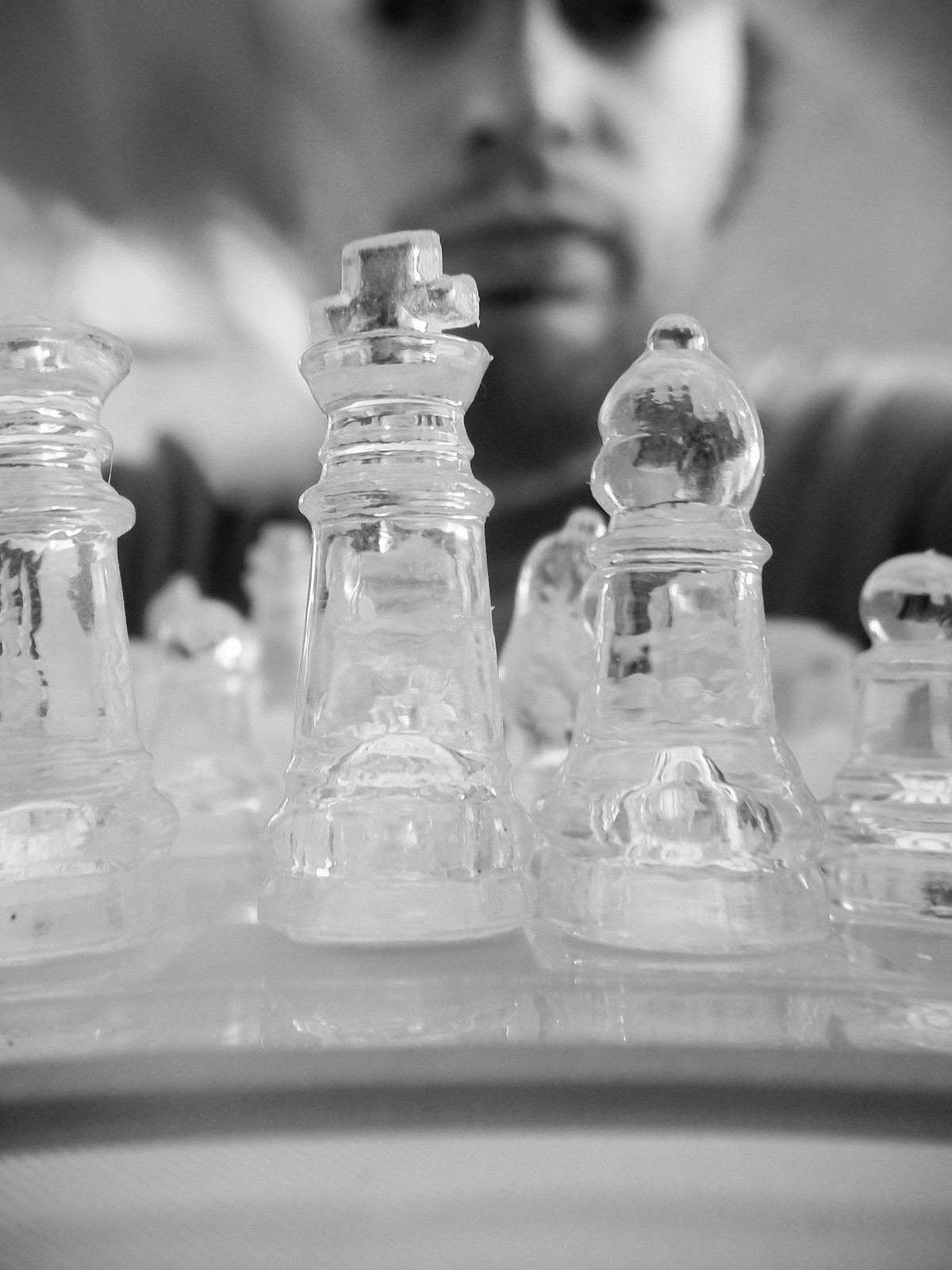This is a black and white close-up photograph of a chess game in progress, capturing crystal clear glass pieces on a glass board. Central to the image, we see the king, easily identifiable by the cross at its top, flanked by the queen to the left and a bishop to the right, distinguishable by its steeple-like top. The rook stands prominently to the far right, with a distinct shape resembling a castle tower, and nearby, a pawn can be noted in the right corner. The chessboard's squares are subtly distinguishable, though not prominent due to the monochromatic color scheme. Behind the luminous pieces looms a blurred male figure, sporting a mustache and goatee, intently focused on the game. His dark shirt contrasts against the lighter backdrop, adding depth to the image. Despite the close-up angle obscuring certain board details, the photograph vividly captures the tension and concentration of the chess competition.